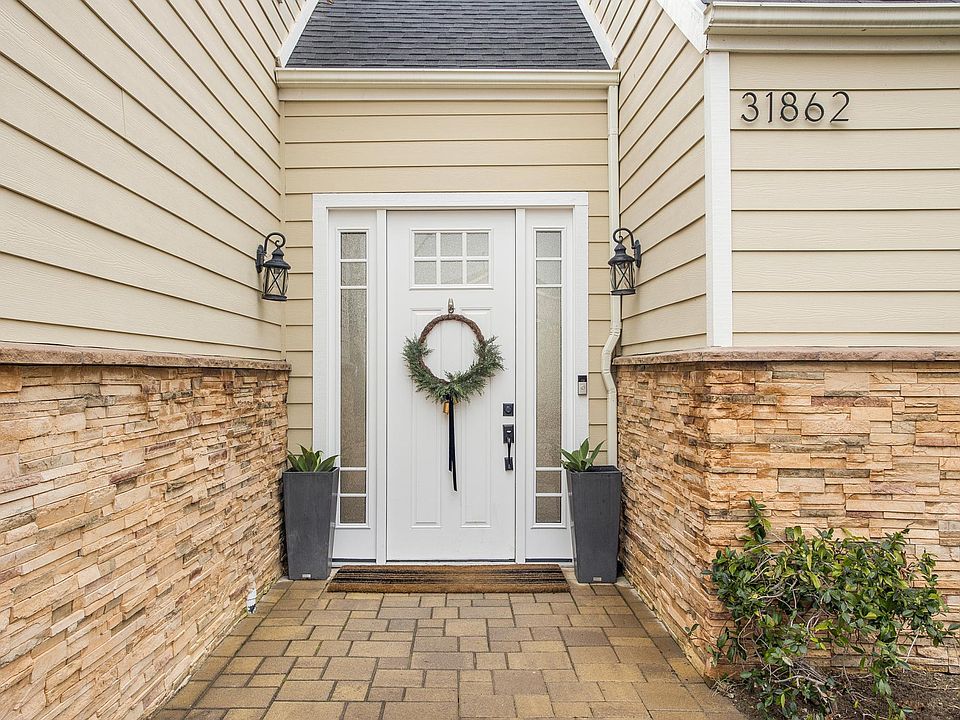In this detailed daytime photograph, the image captures the front entryway of a home with house number 31862. The scene reveals a meticulously maintained approach with a brown stone walkway leading to a white front door, distinguished by a unique grid window pattern formed by six small squares at the top. Flanking the door are two slender windows, known as sidelights. Adorning the door is a round wooden wreath with evergreen branches tied to its bottom half. 

On either side of the entryway, tall black planters host vibrant green plants, while matching black cast-iron lanterns hang from sconces, providing symmetry and charm. The house itself features a lower portion constructed from thin limestone brick, transitioning to tan vinyl siding with white trim above. A small evergreen shrub grows nearby, contributing to the lush, welcoming atmosphere. Underscoring the entrance is a brown-and-black floor mat, complementing the natural tones of the setting. Notably, there is a scraggly looking plant in the lower right-hand corner, adding an element of casual, organic growth to the otherwise orderly appearance.

Overall, this photograph captures the detailed and inviting aesthetic of this home's front exterior, from the well-coordinated decor to the precision of the architectural elements.